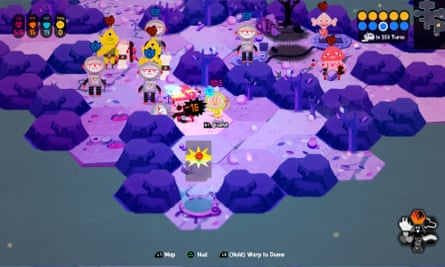This image is a rectangular screenshot from a video game, featuring a mixture of terrain types that include dark purple raised areas and light purple flat regions. These areas form a hexagonal grid across the map, interspersed with blue rocky sections which may be impassable. In the scene, various characters are visible, including a distinct mushroom character with a red polka-dotted hat and others wearing gray helmets. At the top right-hand corner, there is a legend displaying a line of five yellow circles and below them, a line of four blue circles, with a white circle in the third position of the blue row, possibly indicating a specific play. The top left corner shows four small symbols colored red, orange, blue, and yellow. Scattered rocks and pebbles can be seen on the ground, with a bluish tint spreading towards the bottom of the image. There is also some illegible text at the bottom, likely instructions or in-game commentary, alongside a small notification showing "-15". The overall scene has elements of exploration and platforming, consistent with a video game environment.